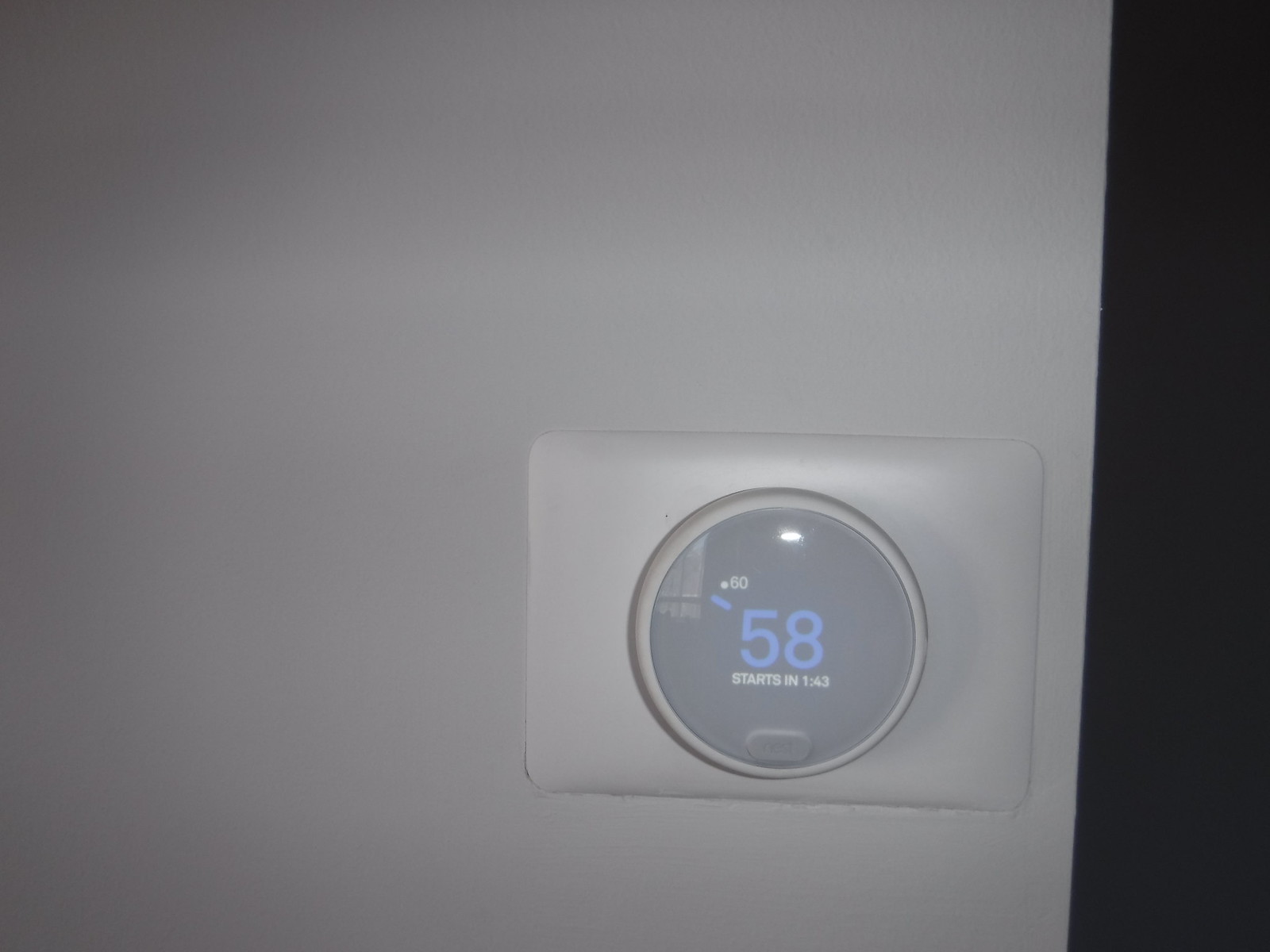This photograph captures a section of a room with a pristine white wall. On the left side of the image, a prominent black bar extends vertically from the ceiling to the floor, possibly indicating an open doorway or hallway entrance. The wall itself is a stark, pure white, though it is not evenly illuminated, resulting in some subtle shadows. 

The focal point of the image is a white plastic thermostat, rectangular in shape, resembling a bar of ivory soap. In the center of the thermostat, there is a circular white control with a protruding glass bubble. Below this circular control, an LCD display is visible, showing the temperature. The display reads the current temperature as "60" in small, white numbers, while the target temperature of "58" is prominently displayed in larger, blue numbers. Beneath this, the text "starts in 1:43" is shown in white, indicating a countdown or timer setting on the thermostat.